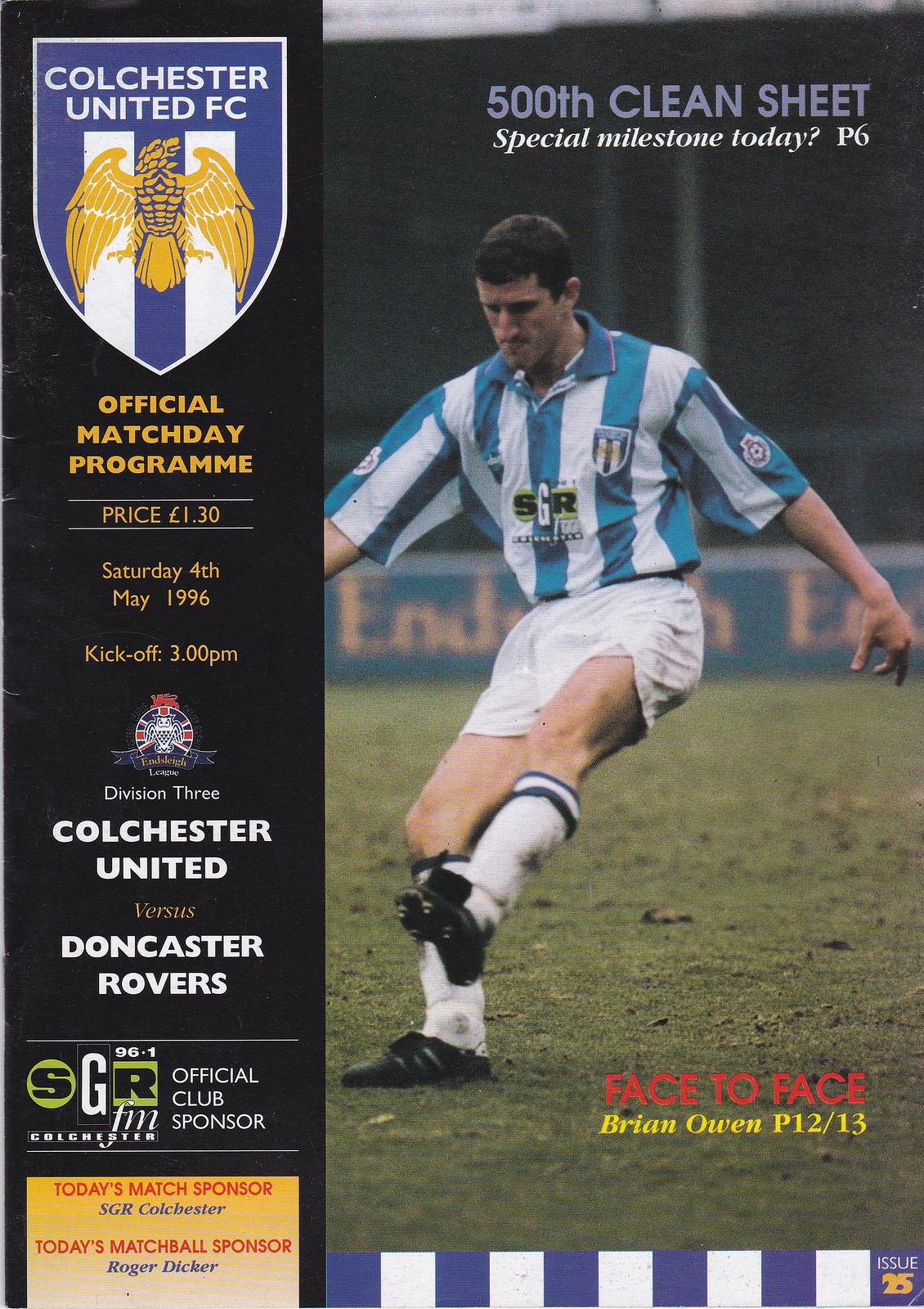This colorful flyer is the official match day program for a Division III soccer game between Colchester United and Doncaster Rovers, held on Saturday, May 4, 1996, at 3 PM. Priced at one British pound and thirty pence, the program features a prominent photograph of a player in action on the right side, wearing a blue and white striped jersey, white shorts, white socks with black trim, and black cleats. Above the player's image, it highlights a significant event: "500th Clean Sheet Special Milestone Today." Additional information includes an article, "Face to Face with Brian Owen," on pages 12-13. The Colchester United FC crest is displayed on the top left, with blue and white stripes and a golden eagle. The program includes various sponsor mentions: SGR Colchester as the official club sponsor and today's match sponsor, and Roger Dicker as the match ball sponsor. The cover also features a blue and white checkered pattern and a black vertical band running from top to bottom on the left side.